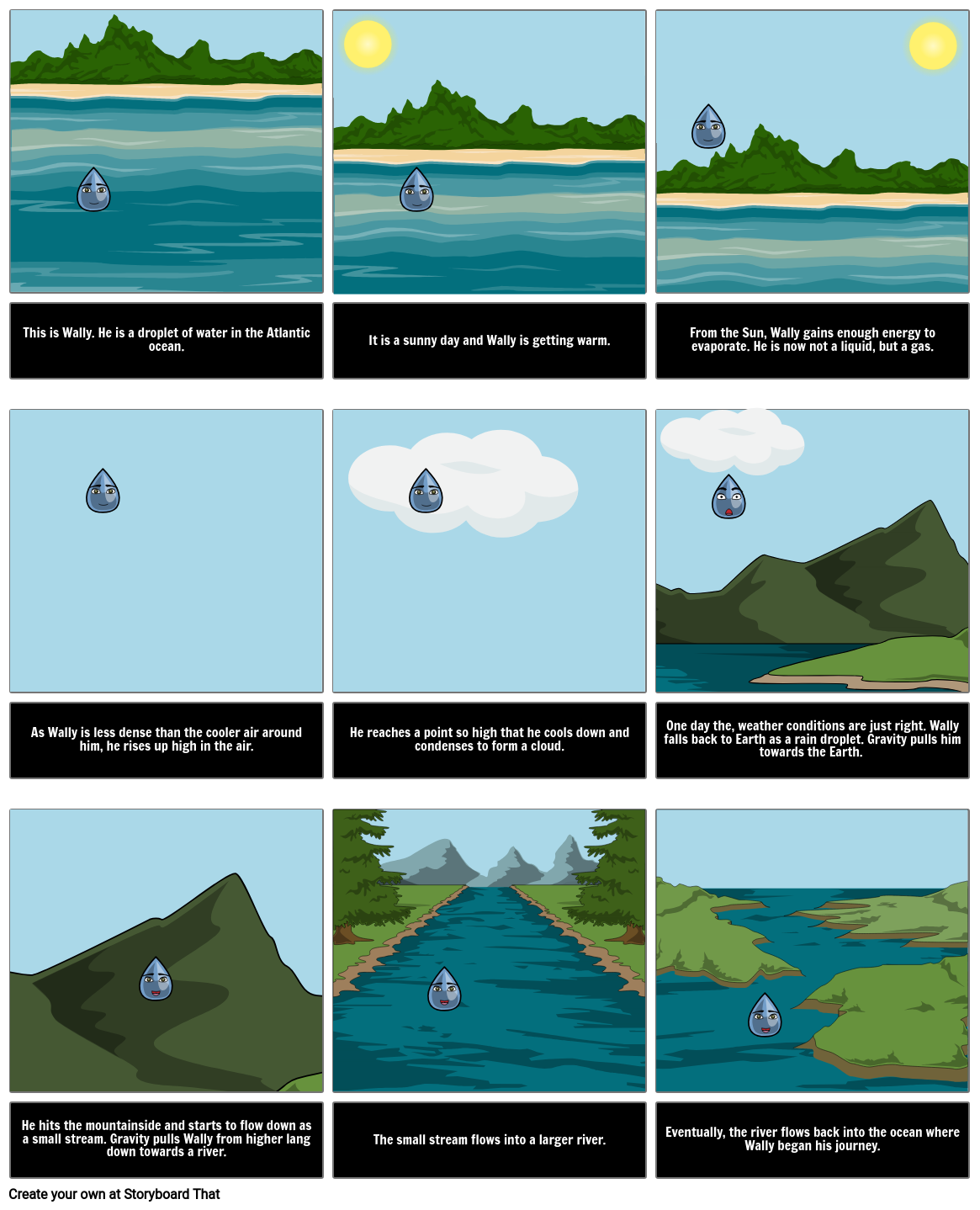This detailed storyboard, divided into nine squares, tells the illustrated journey of Wally, a droplet of water in the Atlantic Ocean. Each panel includes vivid colors, featuring blue skies, green landscapes, and sandy beaches.

In the first panel, Wally the water droplet is falling towards the sea, with majestic mountains and a beach in the background. A subtitle introduces Wally: "This is Wally, he is a droplet of water in the Atlantic Ocean."

In the second panel, Wally is seen hovering just above the water, with the sun shining brightly above the mountains, indicating a sunny day. The subtitle reads, "It is a sunny day and Wally is getting warm."

By the third panel, Wally has risen higher as the sun shifts to the upper right corner. The subtitle narrates, "From the sun, Wally gains enough energy to evaporate. He is now not a liquid, but a gas."

The fourth panel shows Wally in a blue sky, indicating his evaporation process, with the subtitle stating, "As Wally is less dense than the cooler air around him, he rises up high in the air."

In the fifth panel, Wally is shown entering a cloud, and the text explains, "He reaches a point so high that he cools down and condenses to form a cloud."

The sixth panel depicts Wally falling out of the cloud, with mountains and a river in the background. The subtitle reveals, "One day, the weather conditions are just right. Wally falls back to Earth as a raindrop, and gravity pulls him towards the earth."

In the seventh panel, Wally hits a mountain and starts flowing down as a small stream, with the subtitle reading, "He hits the mountainside and starts to flow down as a small stream. Gravity pulls Wally from higher land down towards the river."

The eighth panel shows Wally in a river bordered by trees and mountains. The subtitle notes, "The small stream flows into a larger river."

In the ninth and final panel, Wally is back in the ocean near the shore, concluding his journey. The subtitle reads, "Eventually the river flows back into the ocean where Wally began his journey."

This descriptive storyboard effectively captures every stage of Wally's adventure through the water cycle, from the ocean to the sky, and back again.